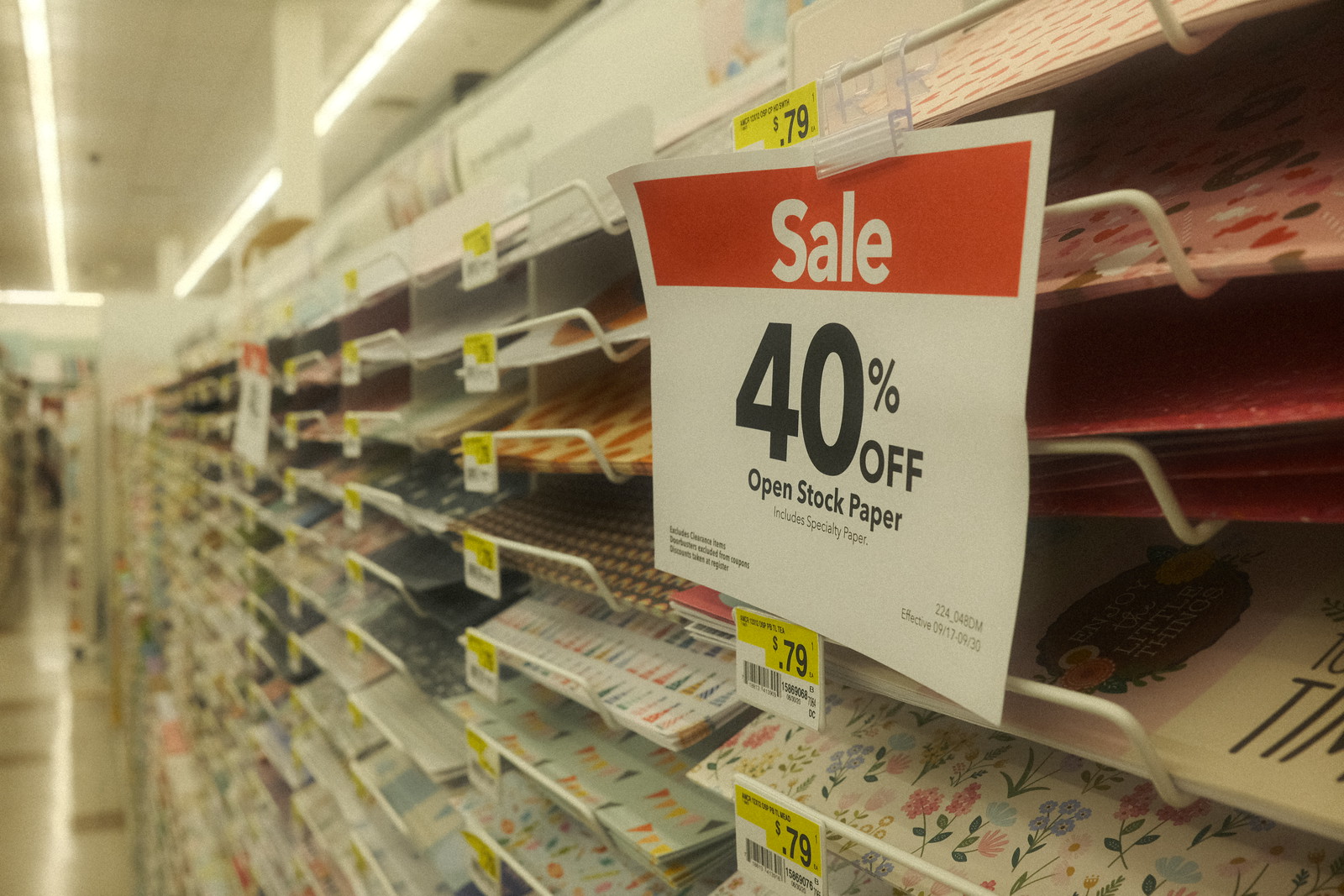In the photo, there is a brightly lit store with a long wall of shelves extending to the back. At the top of the wall, a white piece of paper is prominently displayed, with the text "SAIL" in white lettering against a red background. Below it, another sign indicates a "40% off" sale on open stock specialty paper, though additional text on the right and left sides of the sign is not readable.

The shelves are filled with small trays, each holding different sections of specialty paper that appear to be designed for scrapbooking. The trays are white, coated with a rubbery substance, and supported by wire arms that lift to hold the paper in place. Each tray seems to contain piles of the same type of paper; for example, the tray closest to the viewer holds multicolored floral paper, while another tray above it contains solid red paper. Other trays feature various floral and geometric designs. The comprehensive assortment of paper types spans the entire length of the deep wall, suggesting a well-stocked supply of scrapbooking materials and more.